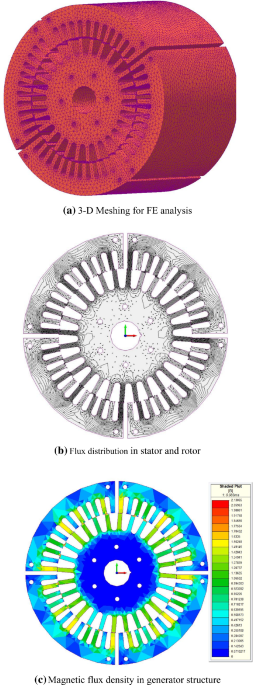The graphic presents three vertically aligned circular diagrams against a white background, each accompanied by explanatory text. The top image, labeled "Figure A," is a 3D depiction of a cylindrical item with a slightly turned perspective, making it appear three-dimensional. It is rendered in hues of dark red, blue, and purple, and features dashed blue lines in two concentric circles. The caption "3D Meshing for FE Analysis" is noted below this image. The middle diagram, "Figure B," shows a head-on view of a silver and gray circular item with black and gray lines emanating from an inner circle towards the outer edge, resembling clock hands. The description below reads "Flux Distribution in Stator and Rotor." The bottom diagram, "Figure C," illustrates the magnetic flux density in a generator structure. This circle is predominantly green, blue, and light blue, accompanied by a graph on the right showcasing a spectrum of colors from dark red to light blue to represent different flux intensities. The detailed caption for this image states "Magnetic Flux Density in Generator Structure."